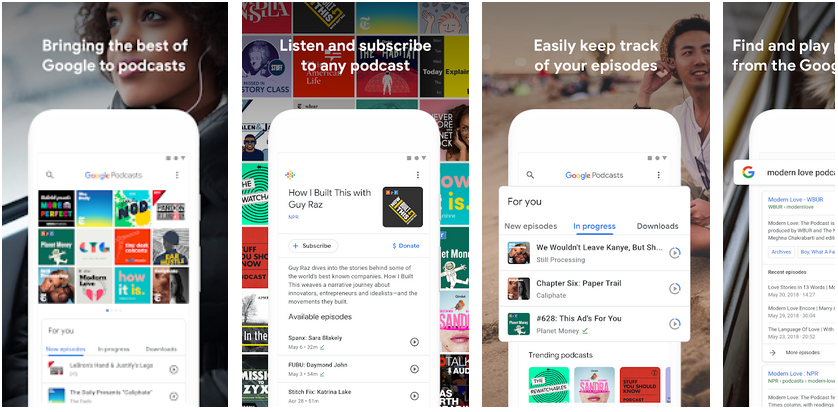This is a set of four images illustrating the features of a Google podcast service. Starting from the left:

1. **Bringing the Best of Google to Podcasts**: The first image showcases a promotional statement emphasizing Google's commitment to enhancing the podcast experience. The background features a close-up image of a woman, presumably enjoying a podcast, highlighting the human aspect of podcast listening.

2. **Listen and Subscribe to Any Podcast**: The second image features an interface where users can listen to and subscribe to any podcast of their choice. There are various podcast titles displayed against a backdrop that includes subtle images of books, suggesting a blend of education and entertainment.

3. **Easily Keep Track**: In the third image, a male figure appears in the upper right corner, and the focus is on an interface that helps users easily keep track of their podcast subscriptions and listening history. This feature is illustrated through a clear and user-friendly layout.

4. **Infinite Play**: The fourth image, though partially cut off, appears to demonstrate a continuous or infinite play feature, allowing the user to enjoy seamless podcast playback. The background includes several images, but due to the cut-off nature, they are not fully visible.

Overall, the four images collectively highlight the various capabilities and features of Google's podcast service, namely its comprehensive access, user-friendly interface, and seamless continuous play feature.